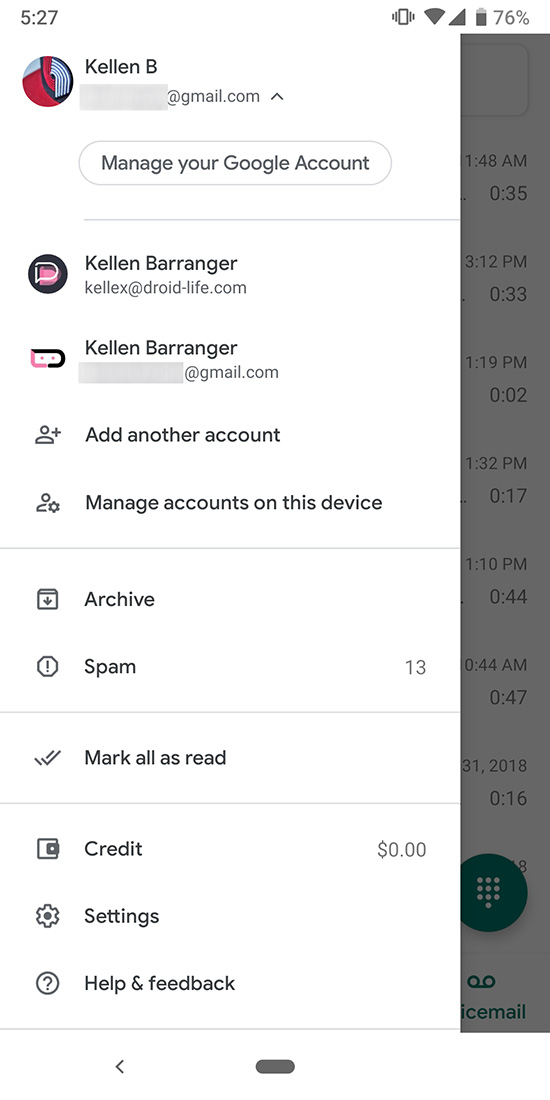In the screenshot, located in the top left corner, the time is displayed as 5:27, while the battery status on the top right corner reads 76%. In the center, there is a small circular profile image dominated by hues of red and a touch of gray, next to which the name "Kellen B." is displayed prominently.

Beneath this, a gray square reveals a partially obscured email address displaying only "@gmail.com". Following that, the text "Manage your Google account" is visible. Below that, the name "Kellen Berenger" appears a second time alongside the email "kellex@droid-life.com", and once more with an obscured email ending in "@gmail.com".

Further options listed include "Add another account" and "Manage accounts on this device", separated by a long gray line. Subsequent options include "Archive" and "Spam," with the latter accompanied by the number 13 to its right. Another long gray line follows, underneath which, the option "Mark all as read" with a check mark is present.

Below this section, a long gray line precedes the "Credit" option, displaying a balance of 0.00 to its right. Further down, there are options for "Settings," "Help and feedback," and at the very bottom, a short black line.